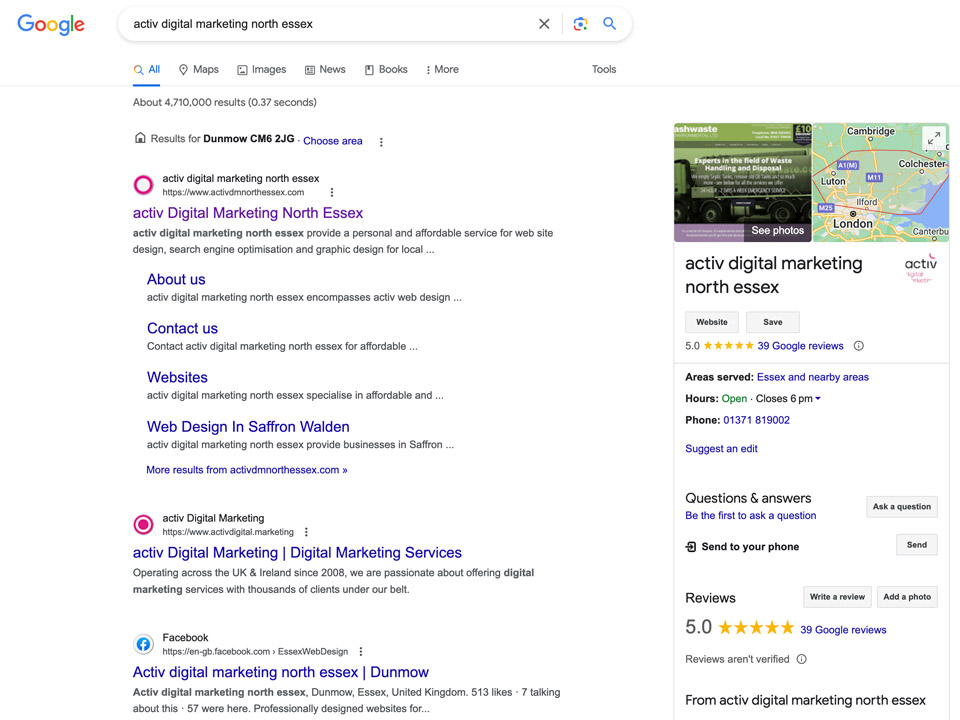In the screenshot captured, the webpage displayed is from Google’s search engine. At the top, displayed in the search bar, is the query "Active Digital Marketing North Exits." Beneath the search bar, tabs labeled "All," "Maps," "Images," "News," "Books," and "More" are visible, each with corresponding icons. The results indicate that there are approximately 4,710,000 results generated in 0.37 seconds.

The primary search result pertains to "Dunmow CM6JG Choose Area." One prominent result is "Active Digital Marketing North Essex," which features a small circular icon to its left. This headline is succeeded by links labeled "About Us," "Contact Us," "Website," "Web Design," and "Safron Walden."

To the right, detailed information about "Active Digital Marketing North Essex" is provided. This includes a map with green and blue areas, indicating regions near water bodies, focusing on London and Cambridge as significant reference points. Accompanying this is a "Website" button that directs to their website, along with a "Save" button.

Additional pertinent details include the service areas listed as Essex and nearby regions, operational hours noting closure at 6 p.m., and a contact phone number: 01371-819-002. The left-hand column reiterates "Active Digital Marketing" and provides a link to their Facebook page, integrated into the search engine results.